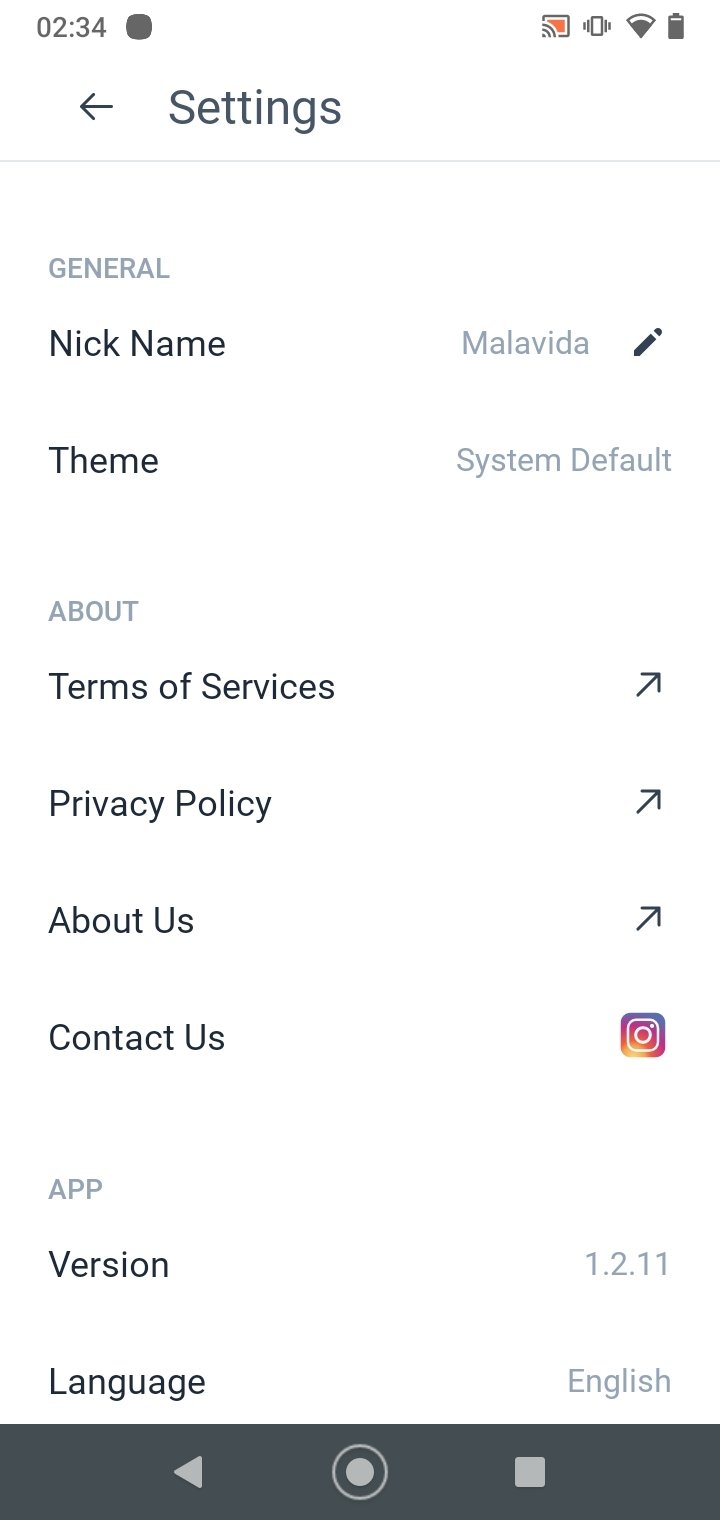The image is a screenshot of an Android phone taken at 2:34 AM, as indicated by the timestamp in the top-left corner. The status bar shows a black square, a Wi-Fi icon that is three-fourths full, and a silent mode indicator. The battery icon also appears to be three-fourths full.

The screenshot features a "Settings" menu, specifically within the "General Settings" section of an unspecified app. At the top of the screen is a back arrow, followed by the "Settings" title. Below it, a subsection titled "Nickname" allows for editing, with the current nickname set to "Malavida". The "Theme" is set to "System Default".

Further down, there are several options including "About", "Terms of Service" (with an arrow indicating a hyperlink that likely redirects to an external web browser), "Privacy Policy", "About Us", and "Contact Us". Interestingly, the "Contact Us" option features an Instagram logo, suggesting that contact can only be made through Instagram, which could be seen as unconventional or suspicious for an app's contact method.

The app version is listed as 1.2.11 and the language is set to English. The overall impression is of a settings interface for a user-focused application, though the restricted contact method through Instagram might raise questions about the app's legitimacy.